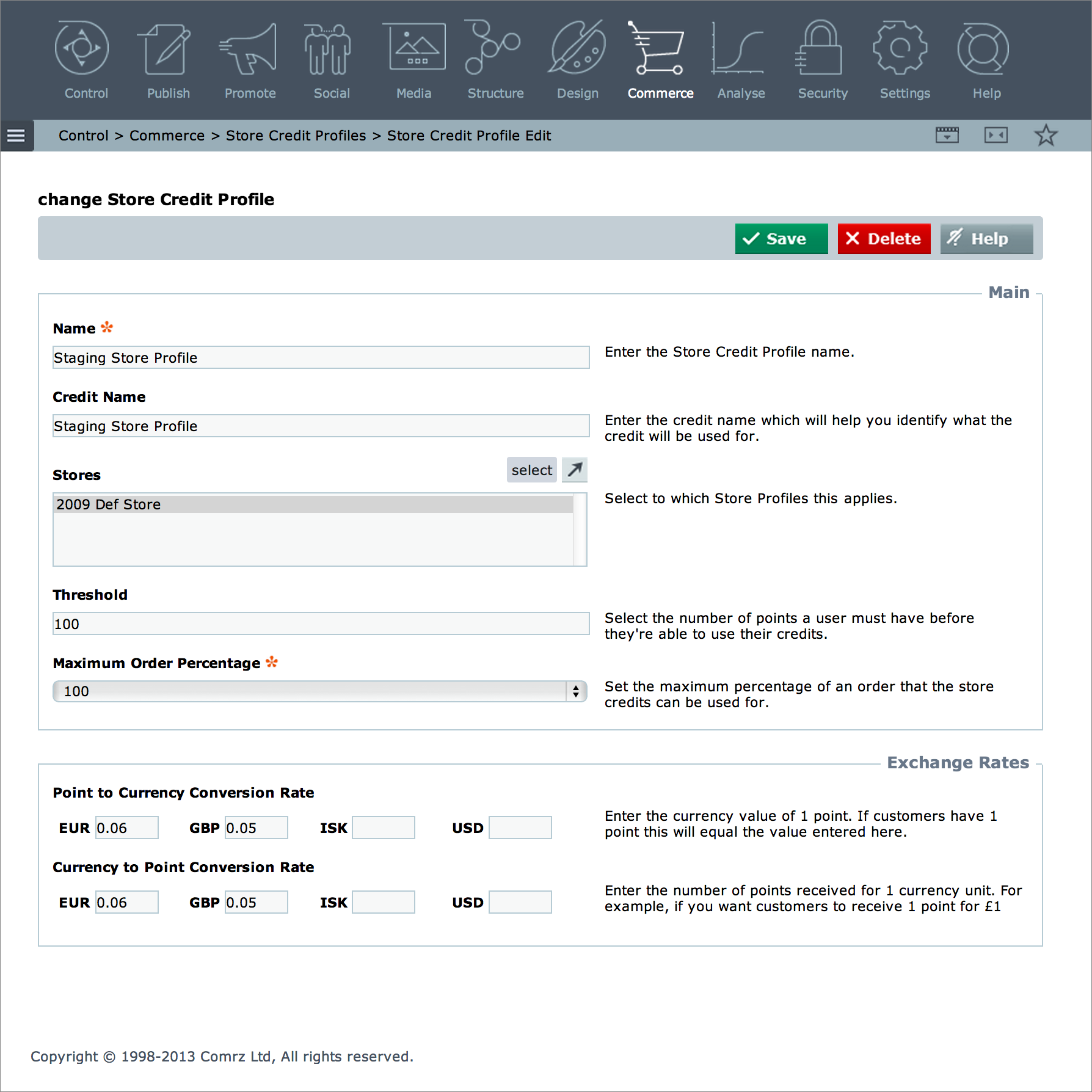The image depicts a screenshot of a web interface with a structured layout.

At the top of the screenshot is a dark blue header that spans the width of the image. This header contains various menu items labeled from left to right: "Control," "Publish," "Promote" (accompanied by the icon of a megaphone), "Social Media" (with an artist's palette and paintbrush icon), "Structure," "Design," "Commerce" (featuring a white shopping cart icon), "Analyze," "Security," "Settings," and "Health."

Directly below the header is a small blue banner, reading from left to right: "Control," "Commerce," "Store Credit Profiles," "Store Credit Profile," and an "Edit" option.

Beneath this banner is a large white page displaying a form titled "Change Store Credit Profile." Situated to the right of this form are three action buttons: a green "Save" button, a red "Delete" button, and a gray "Help" button.

The form itself includes fields labeled: "Name," "Credit Name," "Stores," "Threshold," and "Maximum Order Percentage," providing a comprehensive interface for managing store credit profiles.